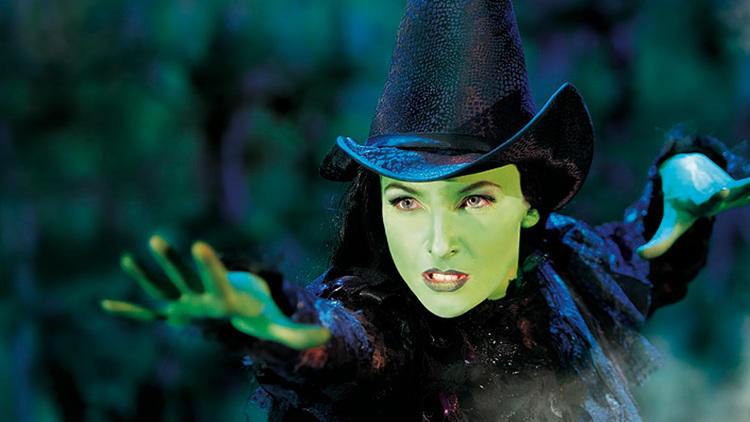The image appears to be a screen capture from a movie or TV show, depicting a woman with green skin, likely playing a witch character. She is positioned slightly to the right of center, facing forward but looking angrily to the left. Her hat is a pointy black or possibly dark purple witch's hat with a texture reminiscent of scales. She has long, black hair and is wearing a flowing black cloak that may have hints of pinks and oranges. Her fingers are spread apart, with her right arm stretched out in front and her left arm pulled back at shoulder height, suggesting she might be casting a spell. The blurred background features mingled colors of dark green, dark blue, and black, possibly hinting at trees or dark plant life.